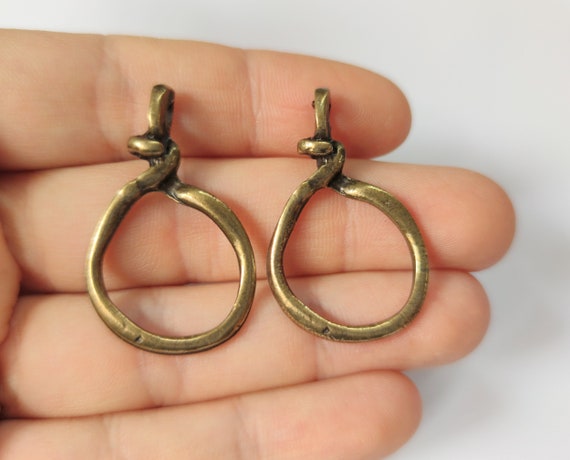The image is a close-up of a Caucasian person's left hand against a white background with subtle grey shadows cast by the fingers. The focus is on the four fingers—index, middle, ring, and pinky—with no thumb in view, extending into the upper portion of the palm. Resting on the open palm are two brass-colored metal objects, resembling vintage hoop earrings, though they lack the components typically used to secure them in the ear. These items have a handmade appearance, with slight variations in size and noticeable wear, including small dents and tarnishing. Each metal loop, about the width of two fingers, twists at the top, which could indicate they are part of a necklace or old machinery parts. The brass objects are centrally positioned on the palm, highlighting their intricate, somewhat rusted details against the soft skin tone.